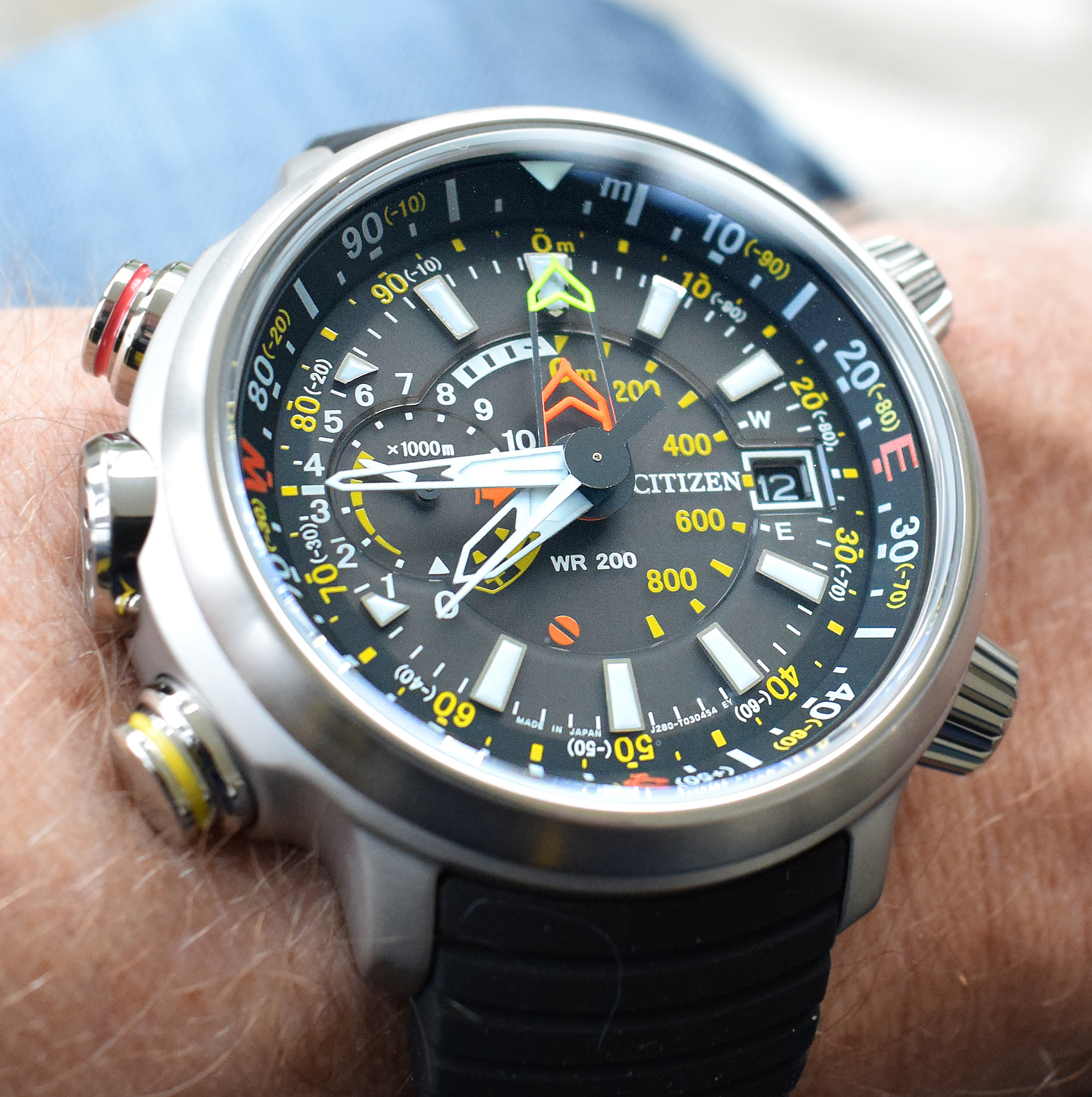The photograph, a close-up square image approximately six inches by six inches, meticulously centers on a large wristwatch. The watch is prominently displayed on the hairy wrist of a Caucasian male, with blonde hairs visible even on the black watch band, though the actual hand and upper arm are not shown. The background, slightly blurred, reveals what appears to be blue jeans and a white area on the right-hand side.

The wristwatch itself commands the viewer’s attention with its intricate and multifaceted design. Encased in a silver border, the circular face of the Citizen brand timepiece features a black background adorned with an array of white, yellow, and red numbers, letters, and various indicators. Along the periphery, a compass feature marks the directions northeast, southwest, while the dial includes gradations for altitudes and speeds, such as 0, 200, 400 up to 800, and a secondary inner circle displaying numbers from 1 to 10 with an "X 1000 M" marking.

Silver buttons along the outer edge are distinctively marked, one with a red line and another with a yellow line, adding to the detailed and intricate nature of the watch. The dark metallic tones inside the face contrast sharply with the lighter silver, further embellishing its detailed and functional aesthetic.